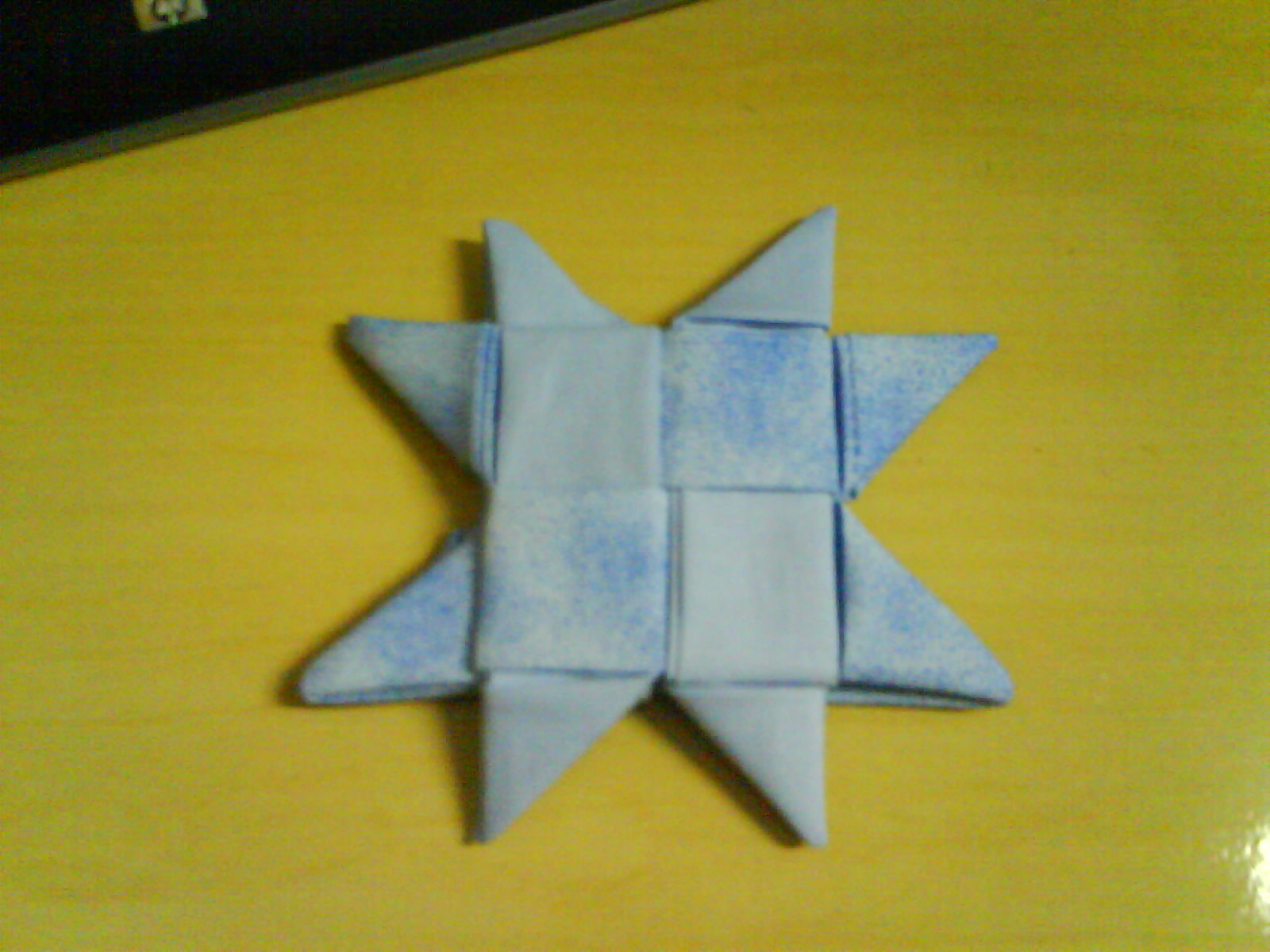The image showcases a light blue paper sculpture with darker blue patches, resembling a combination of a cross and a star with eight points. The sculpture, likely created by a child for a class project or as a craft, is intricately woven to form a central square divided into four smaller squares. Extending from each corner are two points, leading to an overall intricate design that appears symmetrical but not uniformly star-like. This paper creation is carefully placed at the center of a green or light yellow table, which takes up most of the image. The background, blurred and dark, contains an indistinct, gold-colored object that resembles a lock. The indoor setting and the positioning of the sculpture on the table create a focused yet casual composition.